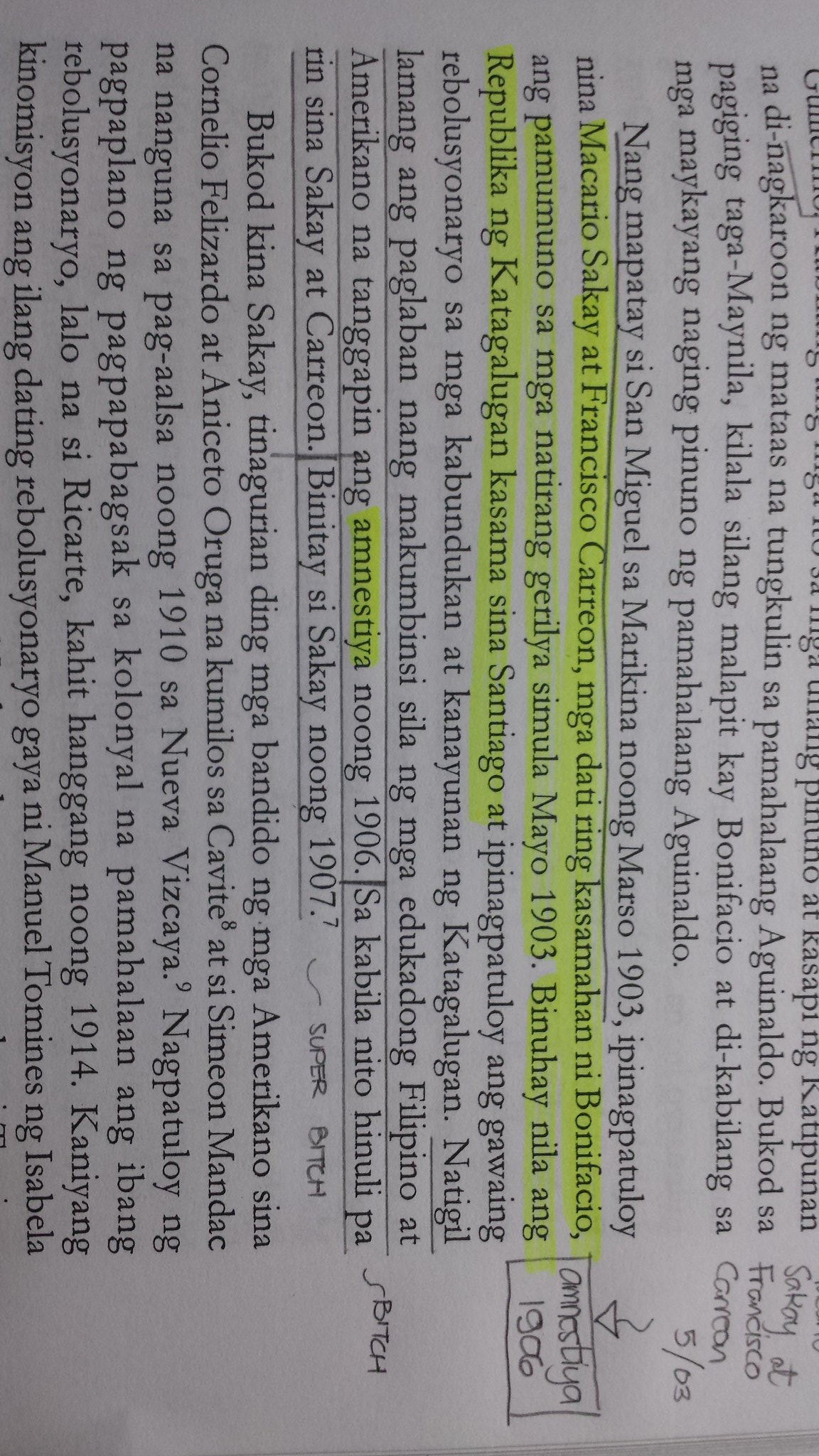The image depicts a sideways page from a book or document, oriented with its text facing horizontally to the right. The text is typed in black on a white background and is written in a foreign language, making it unreadable to English speakers. Sections of the text are highlighted with a marker in a bright color, somewhere between yellow and green. Additionally, some parts of the text are underlined in black ink. Along the right border of the page, there are handwritten notes containing some insulting words about the content of the document. The overall appearance is black and white, save for the highlighted text, giving the page a stark and heavily annotated look.